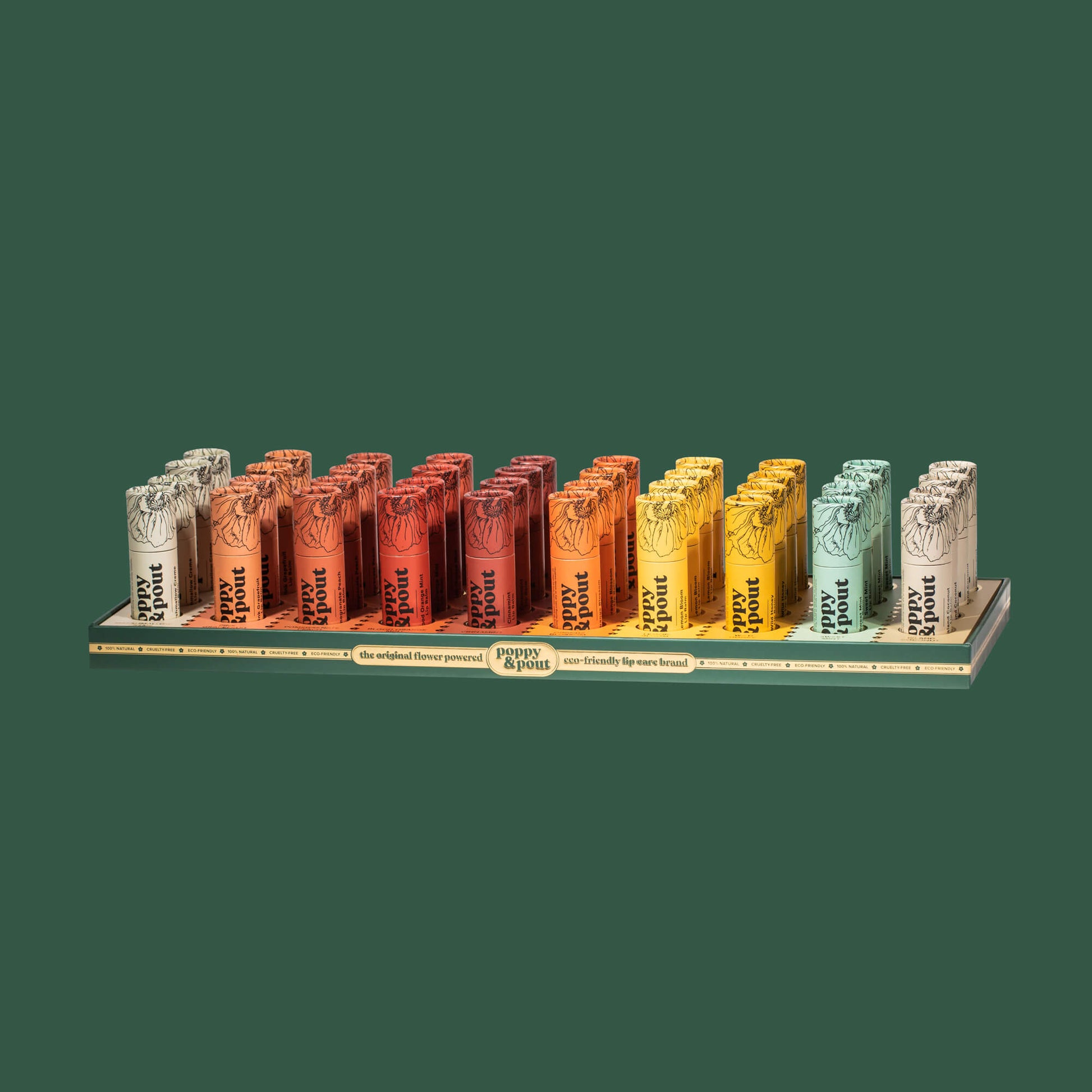This detailed image displays a square display case against a forest green to dark turquoise backdrop, showcasing an assortment of lipsticks, each bearing the text "Poppy and Pout: The Original Flower Powder Eco-Friendly Lip Wear Brand." The lipsticks are neatly arranged in a palette that features 10 distinct rows, each with 4 slots, amounting to a total of 40 lip products. The colors of the lipsticks are varied and vibrant, including shades like white, teal or mint, light yellow, dark yellow, orange, magenta, brown, nude, and different tones of red and pink. This harmonious arrangement is visually appealing, with the array of colors popping against the greenish background, emphasizing the eco-friendly branding of Poppy and Pout.